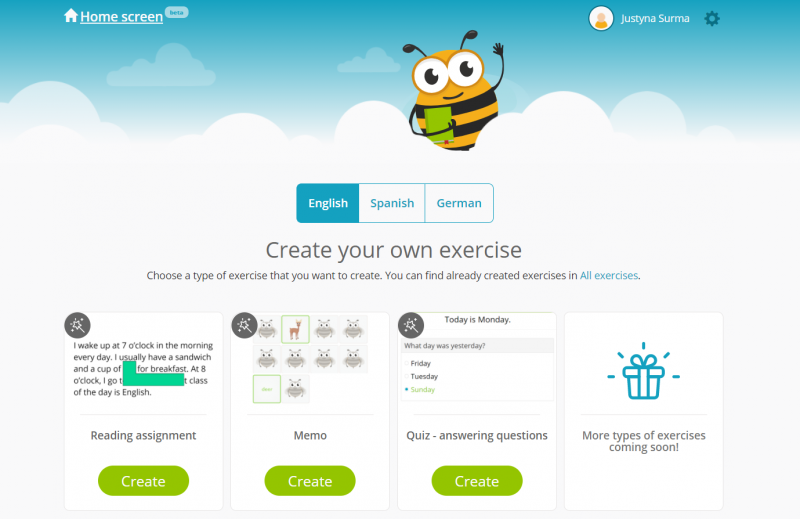This screenshot captures a desktop interface for an educational resource platform in its beta phase. In the top left corner, there's a home screen link labeled as "beta." On the top right corner, a generic profile image is displayed next to the name "Justina Surma," accompanied by a settings gear icon. 

The background of the top third of the page features a sky with clouds, adding a whimsical touch. A friendly bee is illustrated waving and holding a green book, giving the interface a playful element. Below this, three language tabs are visible: English, Spanish, and German.

Under the language tabs, there is a section prompting users to create their own exercise, stating, "Choose the type of exercise that you want to create." It suggests that users can find pre-made exercises by clicking on a link labeled "All Exercises."

Further down, the interface is organized into four columns of boxes for different types of exercises. The first box is for a "Reading Assignment" with a green "Create" button. The second box, labeled "Memo," also includes a green "Create" button. The third box is for "Quiz - Answering Questions," similarly featuring a green "Create" button. The final box displays an image of a present and indicates that "More types of exercises coming soon."

This detailed layout allows users to easily navigate and create a variety of educational exercises on the platform.